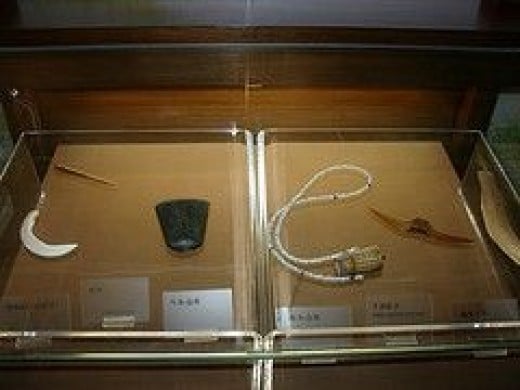In this image, there are two display boxes or specimen boxes positioned side by side, each containing various artifacts protected by glass covers. The overall scene is somewhat blurry, making the details of the items challenging to discern clearly. 

In the left display box, three items are visible. The first is a white U-shaped object resembling a narrow sickle or a moon shape. Above this U-shaped item is a long, pointy object, potentially a pencil or a small stick. The third item in this box is a small, solid black item that might remind one of a tiny trash can but is not one; it could possibly be something like a cup holder.

The right display box contains three more items. The first item looks like a long white necklace, potentially made of beads, possibly attached to a small rectangular beige object. The second item in this case appears to have a resemblance to a bat or a small stingray, with a wing or fin-like structure on either side. The final item is somewhat curved and brown with a darker center, perhaps indicating some sort of crafted artifact.

Each item rests on a beige surface within the display boxes, accompanied by cue cards that likely provide descriptions or names of the items, though the text on the labels is hard to read. The display cases appear to be part of an indoor exhibit, possibly in a museum, and a metal bar runs in front of the cases, suggesting a barrier to prevent close contact with the items on display.